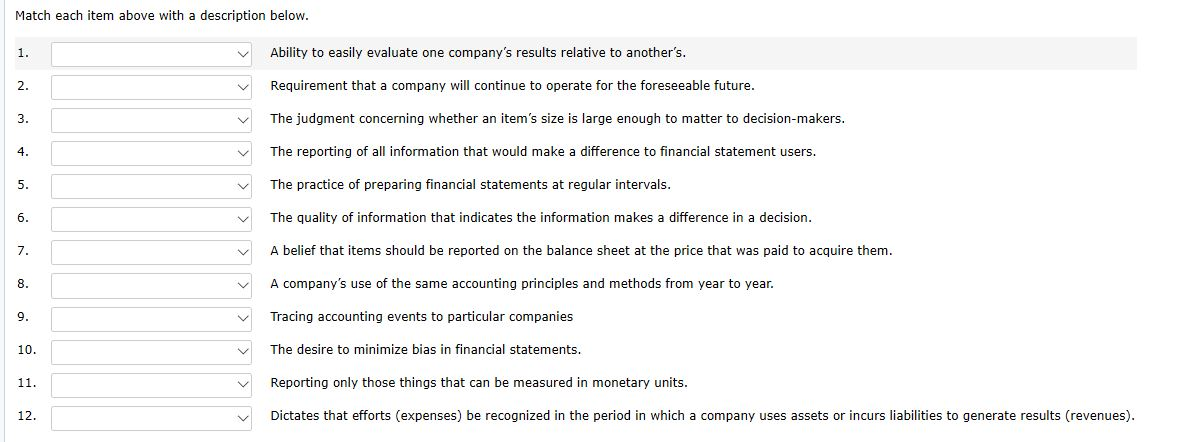**Caption:**

This image features a horizontal screenshot depicting a black and white interface, likely from a quiz, test, or evaluation, related to accounting principles. The screen lacks any colorful elements or icons, establishing a straightforward, no-frills appearance. At the top, the instruction prompts, "Match each item above with the description below." Below this header, there are 12 numerical descriptions, each accompanied by an empty text box intended for user input. 

- **Number 1:** "Ability to easily evaluate one company's results relative to another's."
- **Number 2:** "Requirement that a company will continue to operate for a foreseeable future."
- **Number 3:** "The judgment concerning whether an item's size is large enough to matter to decision makers."
- **Number 4:** "The reporting of all information that would make a difference to financial statement users."
- **Number 5:** "The practice of preparing financial statements at regular intervals."
- **Number 6:** "The quality of information that indicates the information makes a difference in a decision."
- **Number 7:** "A belief that items should be reported on the balance sheet at the price that was paid to acquire them."
- **Number 8:** "A company's use of the same accounting principles and methods from year to year."
- **Number 9:** "Tracing accounting events to particular companies."
- **Number 10:** "The desire to minimize bias in financial statements."
- **Number 11:** "Reporting only those things that can be measured in monetary units."
- **Number 12:** "Dictates that efforts (expenses) be recognized in the period in which a company uses assets or incurs liabilities to generate results (revenues)."

The current item in focus is subtly highlighted in light gray. Clearly, this is an assessment tool aimed at testing knowledge of fundamental accounting concepts.